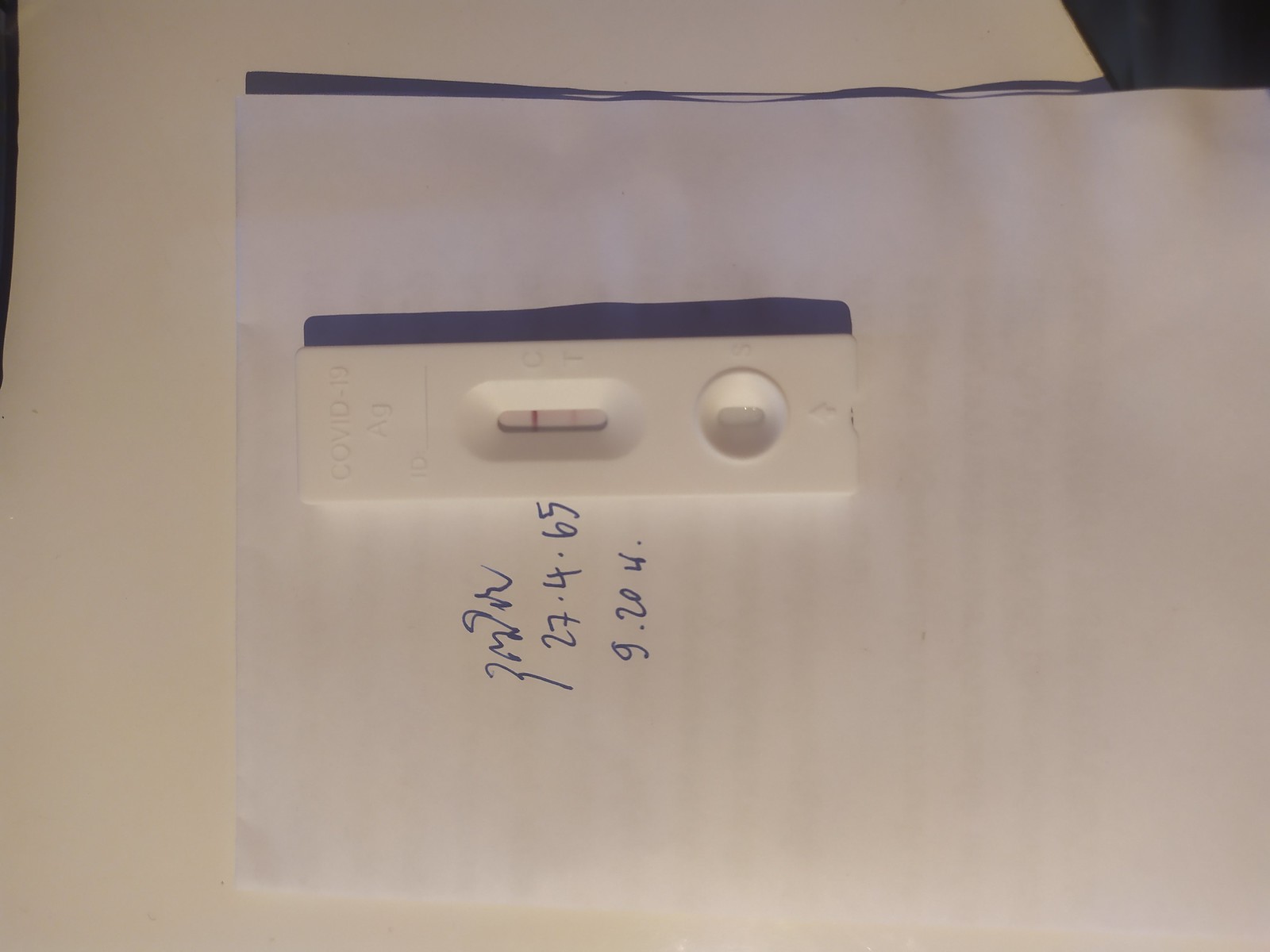The image depicts a partial piece of white paper, either cut or torn in half, lying sideways rather than upright, giving it a slightly crooked appearance. The paper is partially covered in blue ink scribbles, making the writing undiscernible. Notably, there is a date written as "27.4.65," likely referring to April 27th, 1965. Below this date, another set of numbers appears, "9.20.4," whose significance is unclear.

Attached above the handwritten notes is a rectangular piece of plastic with a small indentation. Inside this indentation, a dark red bar is prominently visible. The plastic piece bears printed text, including "COVID-19" and "AG," indicating that it is related to a COVID-19 antigen test.